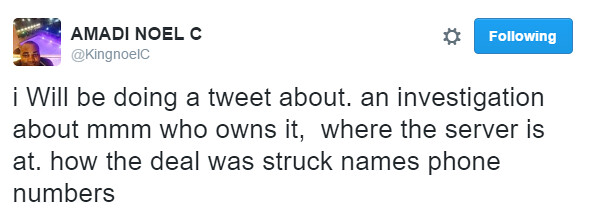This image is a screenshot of a tweet by Amadi Noel C (@KingNoelIC) captured on the social media site Twitter. Clearly visible are the "Following" button and a gear icon at the top right, indicating account settings. The background of the screenshot is predominantly white or transparent. Amadi's profile picture, situated in the lower quadrant, features a black man, possibly in front of a backdrop that hints at music or a pool view, although this is not the main focus.

The tweet text reads: "I will be doing a tweet about an investigation about who owns it, where the server is at, how the deal was struck, names, phone numbers." Though the tweet lacks specific context, it suggests a forthcoming detailed investigation likely about some server, indicating potential investigative interests, possibly in PI work.